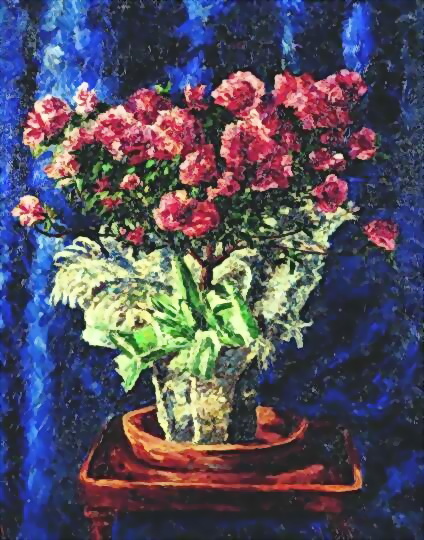The painting depicts a striking and dramatic flower arrangement set against a royal blue background with deep, shadowy folds of a curtain. At the center, a shallow, clear glass container sits on a circular brown plate atop a small wooden square table. Emerging from the container is a vibrant bouquet of pinkish, reddish flowers, likely carnations, all bunched together in various sizes. Interspersed among the flowers are small green leaves adding contrast to the composition. The overall texture and style of the painting impart a hazy, blurred effect, enhancing the dramatic intensity further. The background's bold blue and black hues, reminiscent of a heavy drape, set a dramatic stage for the bright and vibrant floral arrangement, culminating in a visually striking piece of art.